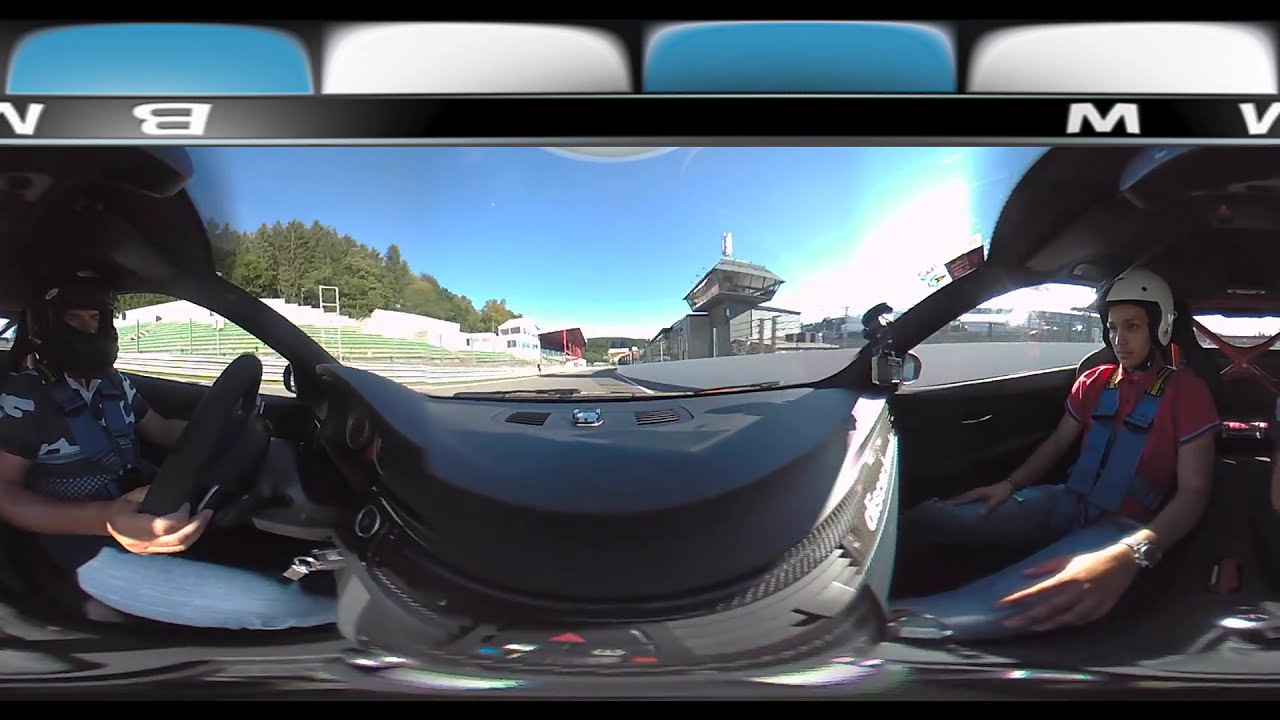This horizontal rectangular image, taken with an unusual camera lens, appears highly distorted, making it challenging to discern exact details. It prominently features a car, with two individuals seated inside, wearing crash helmets and jeans. The person in the passenger seat is positioned on the right, while the driver is on the left. Above them, a dark border contains lettering; on the right side, the text is right side up, whereas on the left side, it is upside down. Additionally, four curved rectangles—two blue and two white—are visible above the border. Between the occupants of the car, a background structure resembling a ramp is evident, hinting at a racing environment. This impression is reinforced by the presence of what looks like bleachers, suggesting that the scene is set in a location where automobiles, likely racing cars, would be driven. The distorted lens effect makes the automobile dominate the lower portion of the visual field.